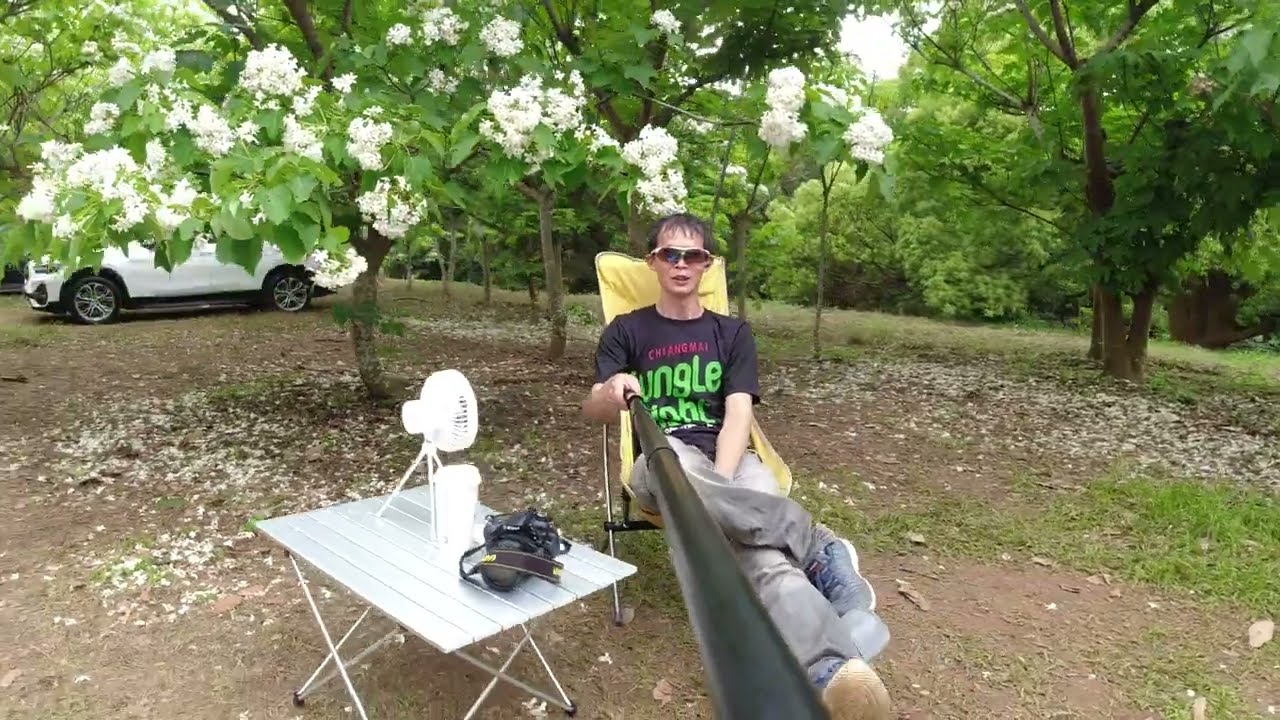In this vibrant outdoor scene, a boy with black sunglasses reclines in a yellow folding camp chair. He wears a black t-shirt with green and red lettering, possibly reading "Jungle Chi-Ik-Meh," along with gray jeans and blue tennis shoes. His dark hair and relaxed demeanor suggest a leisurely moment. He holds a black object, thick enough to resemble a pole, potentially a selfie stick with a cell phone attached. 

Next to him is a folding side table bearing a black camera with a yellow strap and a white fan, indicating he plans to stay awhile. Surrounding him is a lush green environment, with a leafy tree adorned with white flowers behind him, its petals scattered on the ground hinting at springtime. In the distance, a white car, possibly an SUV, is visible in the left corner of the picture against the backdrop of green trees and bushes, providing a serene and homely atmosphere.